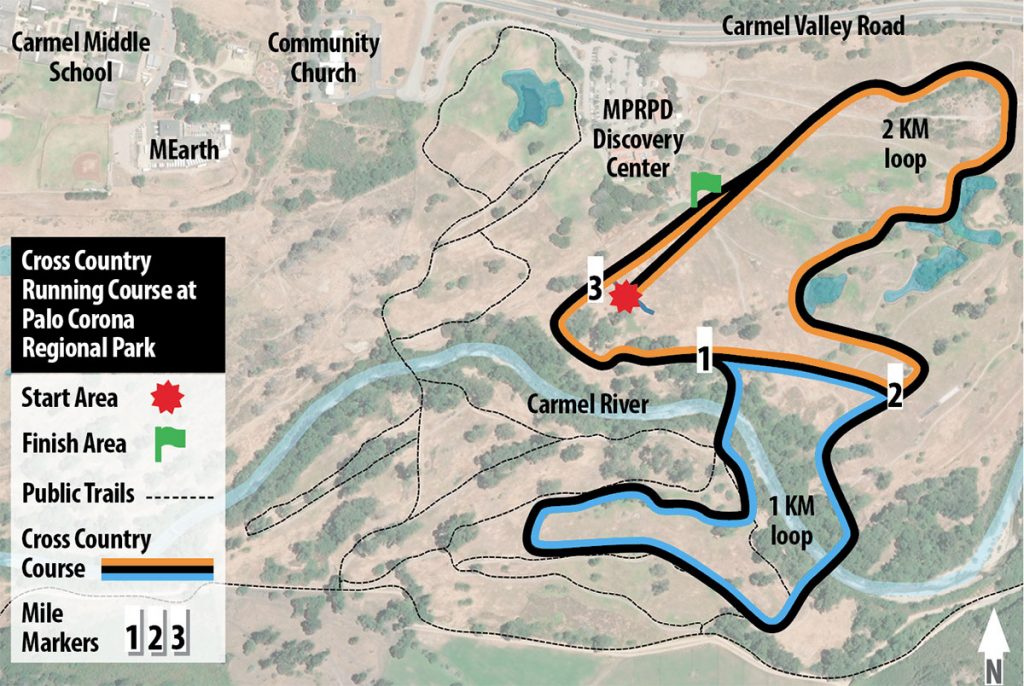The image is a rectangular aerial map of Palo Corona Regional Park, illustrating a cross-country running course. It prominently features two distinct loops of the course, the first loop highlighted in blue and the second in orange. The map includes significant details such as mile markers labeled 1, 2, and 3, and surrounding roads and landmarks. In the top right corner, "Carmel Valley Road" is clearly marked, with the "MPRPD Discovery Center" positioned just below it. To the left, notable locations including the "Community Church," "Me Earth," and "Carmel Middle School" are identified. The bottom left corner of the map contains a legend within a black box with white text, explaining various symbols: a red star for the start area, a green flag for the finish line, dashed lines for public trails, and a black line with either blue or orange markings for the cross-country course. The public trail, forming an extensive path, is shown to the left of the cross-country course, while labels such as "Carmel River" further enrich the map's detailed presentation.